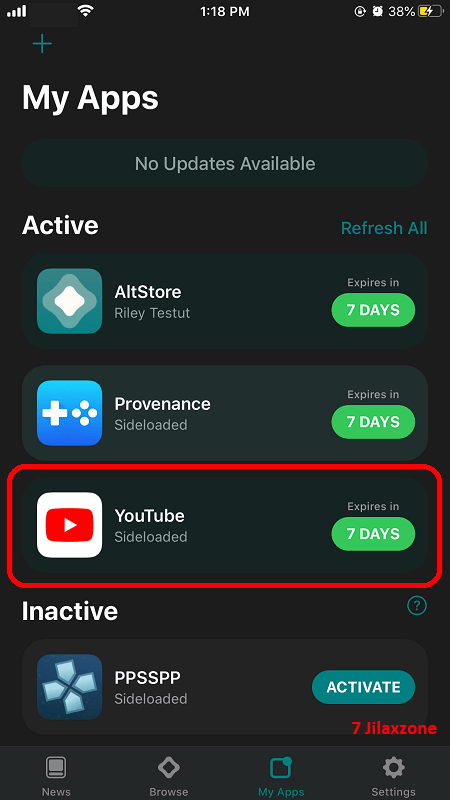The screen displays a detailed summary of the device's status and app information on a black background. The time is 1:18 p.m., and Wi-Fi and data signals are fully active. The battery level is at 38%, with no app updates available. An alarm is also set on the device. 

Highlighted sections include both active and inactive apps. The active apps listed are AltStore, Provenance, and YouTube, all of which are set to expire in seven days and are side-loaded. In the inactive category, PPSSPP appears, having the label 'inactive' next to it. There is an option to refresh all apps.

Notably, YouTube has a red border around it, indicating it was recently interacted with or clipped on. The overall display maintains a consistent dark background, with the text and various options subtly differentiated to highlight their status.